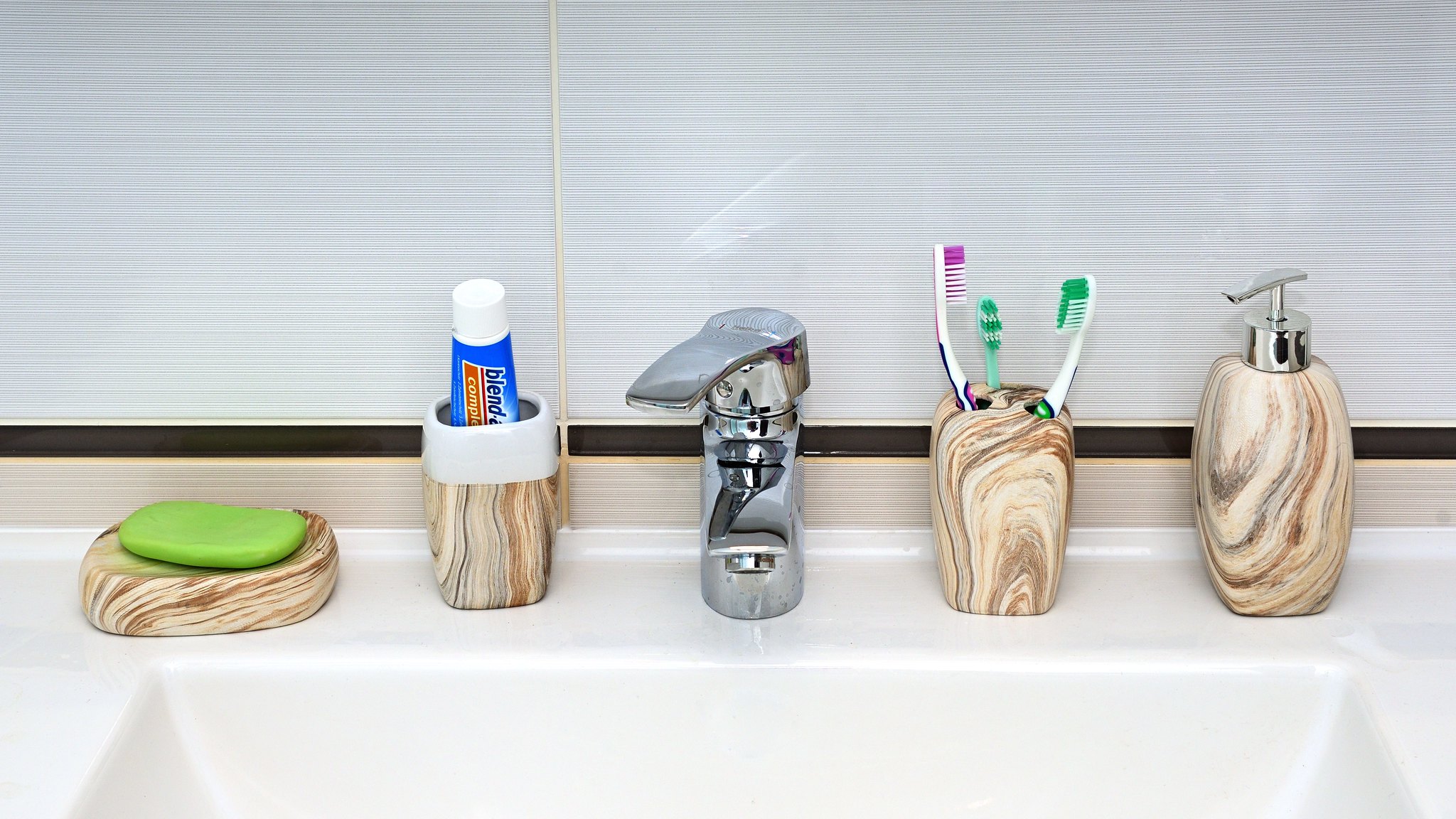A meticulously framed close-up shot of an elegant bathroom sink captures the essence of modern luxury. The large white marble countertop harmonizes with a sleek stainless steel faucet featuring a single-handle design for hot and cold water. To the left of the faucet, a contemporary container set in a natural wood and white marbled pattern holds various items. One canister contains a green bar of dish soap, while another serves as a toothpaste holder with a tube of "Blend Complete" toothpaste visibly protruding. On the right side of the faucet, a matching container holds three toothbrushes in purple, white-and-green, and light green hues. Adjacent to this, a sophisticated soap dispenser made from the same marbled wood and topped with a stainless steel pump completes the arrangement. The background features an architectural, textured wall paneling, adding to the bathroom's refined aesthetic. The entire scene is impeccably clean, bathed in bright light, highlighting the thoughtful design and immaculate condition.